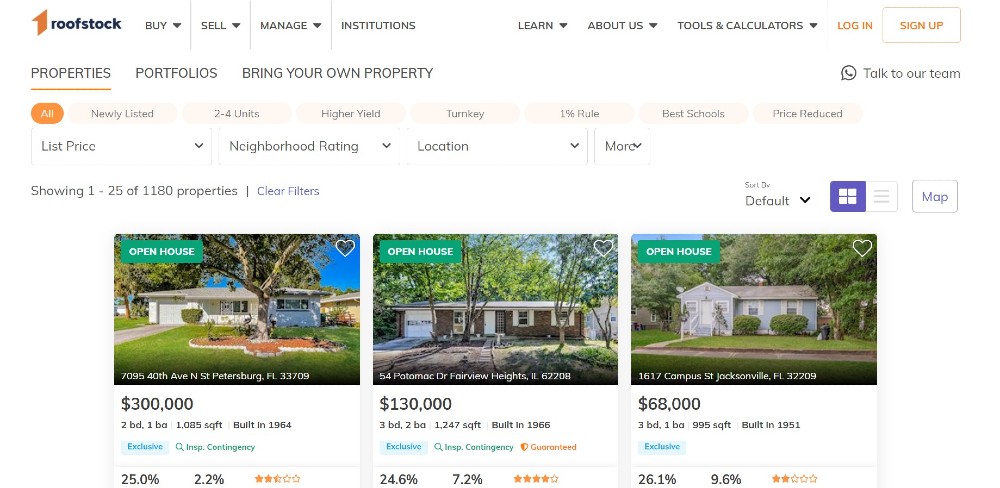The image displays a website named "Roopstock," evident from the label in the top left corner. The webpage showcases three large, single-level house properties prominently in the middle section. Each property is surrounded by lush greenery, with two homes featuring expansive grass fields in front. These homes are accompanied by photographs, detailed with the price, star rating reviews, number of bedrooms and bathrooms, square footage, and the year each house was built. The top right corner of the webpage contains buttons for "Login" and "Sign Up." The website's backdrop is white, while the text throughout the page is rendered in black. Overall, the snapshot captures a clean and detailed real estate listings page on Roopstock, presenting essential property information effectively.